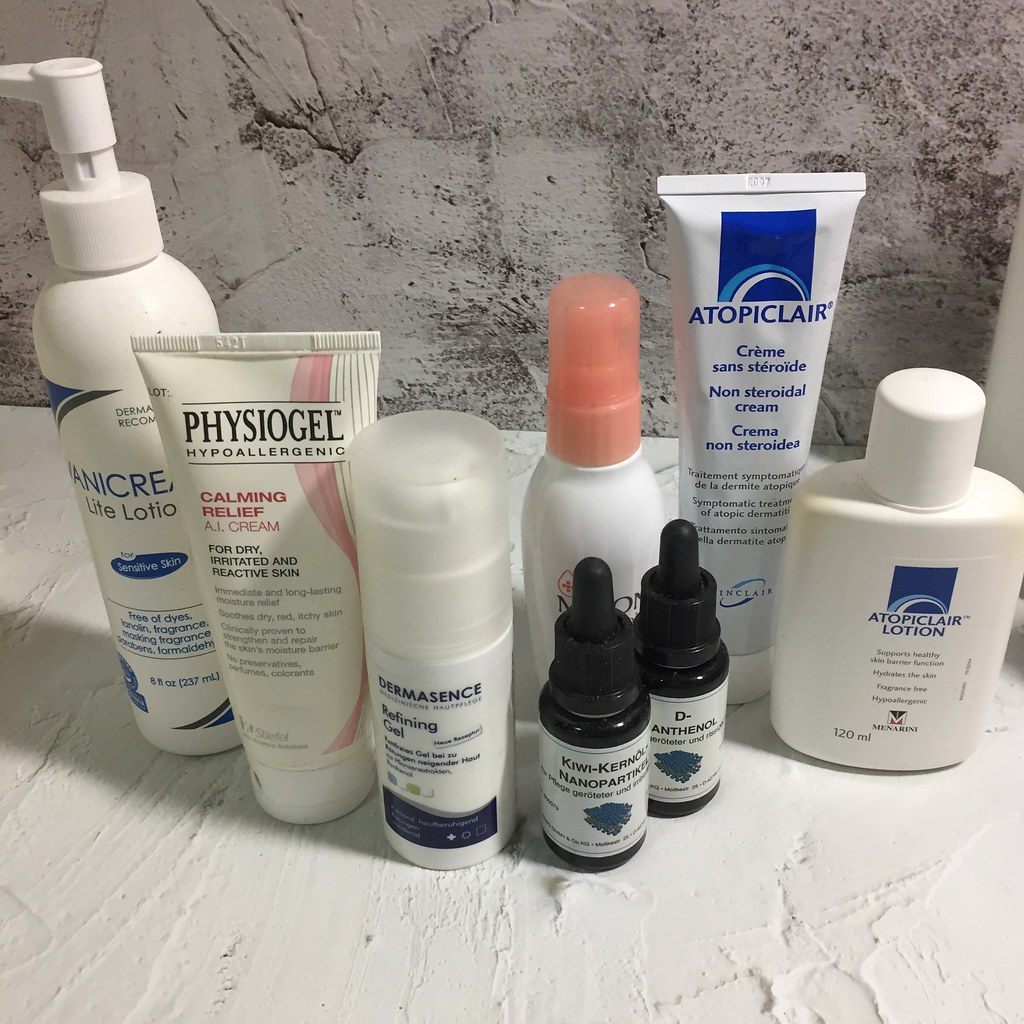The photo, taken indoors, appears to capture a bathroom setting, likely inside a shower area. The backdrop consists of a sleek, gray granite wall that complements the white, textured countertop below. Arranged on this countertop is an assortment of skincare products. Prominently featured are a bottle of Atopic Clear Lotion and a tube of Atopic Clear Non-Steroidal Cream. Two smaller bottles with squeeze tops, labeled "Kiwi something nanoparticle," suggest they are some form of drops. Additionally, there is a bottle of Dermasense Refining Gel, a tube of Visogel, and a container of Hypoallergenic Calming Relief AI Cream, specifically formulated for dry, irritated, and reactive skin. Completing the array is another bottle of lotion designed for sensitive skin. All these items are neatly lined up on the countertop, illustrating an elaborate skincare routine setup within the bathroom space.